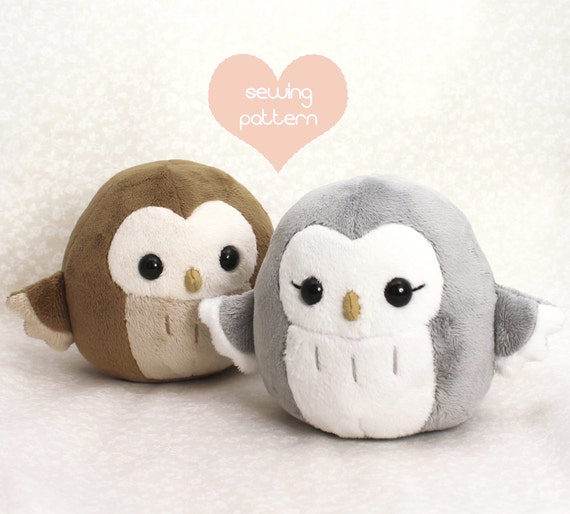In this detailed image, two plush owl toys are featured on a soft, textured cream-colored background with a subtle flower pattern, enhancing a cozy, handmade feel. The gray owl, positioned in the front center, has a white belly and face with additional eye accents resembling eyelashes, giving it a slightly whimsical expression. Behind it sits a taupe-brown owl, which also has a white face and a lighter tan belly and wing accents. Both owls are adorned with black eyes and little yellow beaks. Above the duo, a light pink heart graphic contains the white text "sewing pattern" in a rounded, all lowercase font, indicating that this image represents the end result of a sewing pattern for crafting these plush toys.